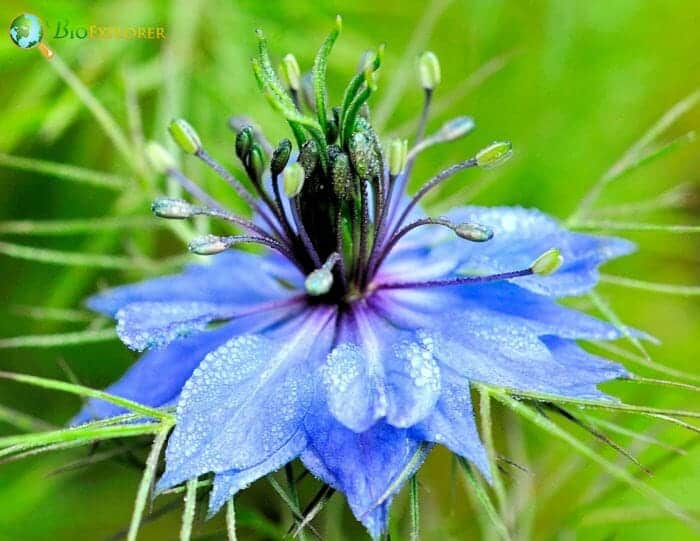This vibrant, close-up nature photograph captures an exotic flower at its most detailed. Central to the image, the petals of the flower display a mesmerizing gradient of blues, from deep navy to sky blue, and hues of lavender and violet. Each delicate petal is adorned with droplets of dew, adding to the flower's refreshing allure. The focus intensifies towards the center where the petals transition into intricate pistils, showcasing colors from purple to green, with some tips appearing almost black.

The background, though blurred, complements the scene with its bright green tones, suggestive of long grass blades, bringing depth and context to the flower's natural habitat. Strings of petals also feature an array of colors—purple, green, and cream—adding to the exotic and vivid appearance of the flower.

In the top left corner, the text "Bio Explorer" accompanied by a globe icon marks the image, hinting at its scientific or exploratory theme. This photograph, set outdoors, captures the essence of nature's intricate beauty through its stunning close-up detail.